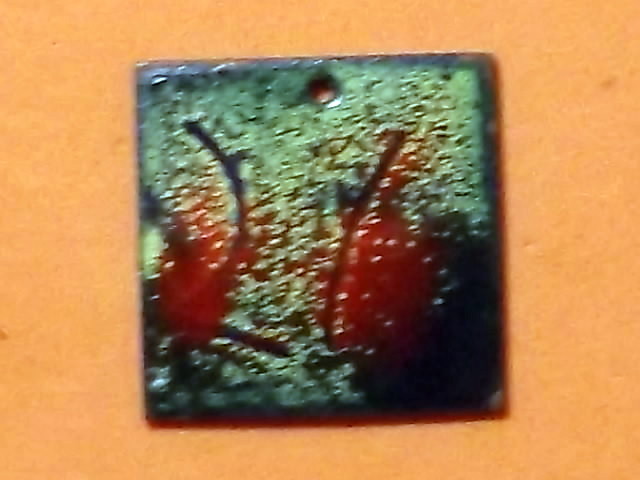The image depicts a decorative square tile, likely made of clay and featuring a tiny hole at the top, possibly for hanging with a string or for affixing to a surface with a nail or screw. The base color of the tile is brown, overlaid with green and textured detailing, along with some dark blue tinges. The detailed design includes vertical, curved lines and red elements that resemble cherries or abstract shapes with curved stems. The picture is slightly blurry, suggesting it was taken in haste. The background is an orange, likely indicating the tile is resting on an orange table or surface rather than being mounted. The overall appearance suggests an old-fashioned, blistered metal look, though it is probably crafted from clay.